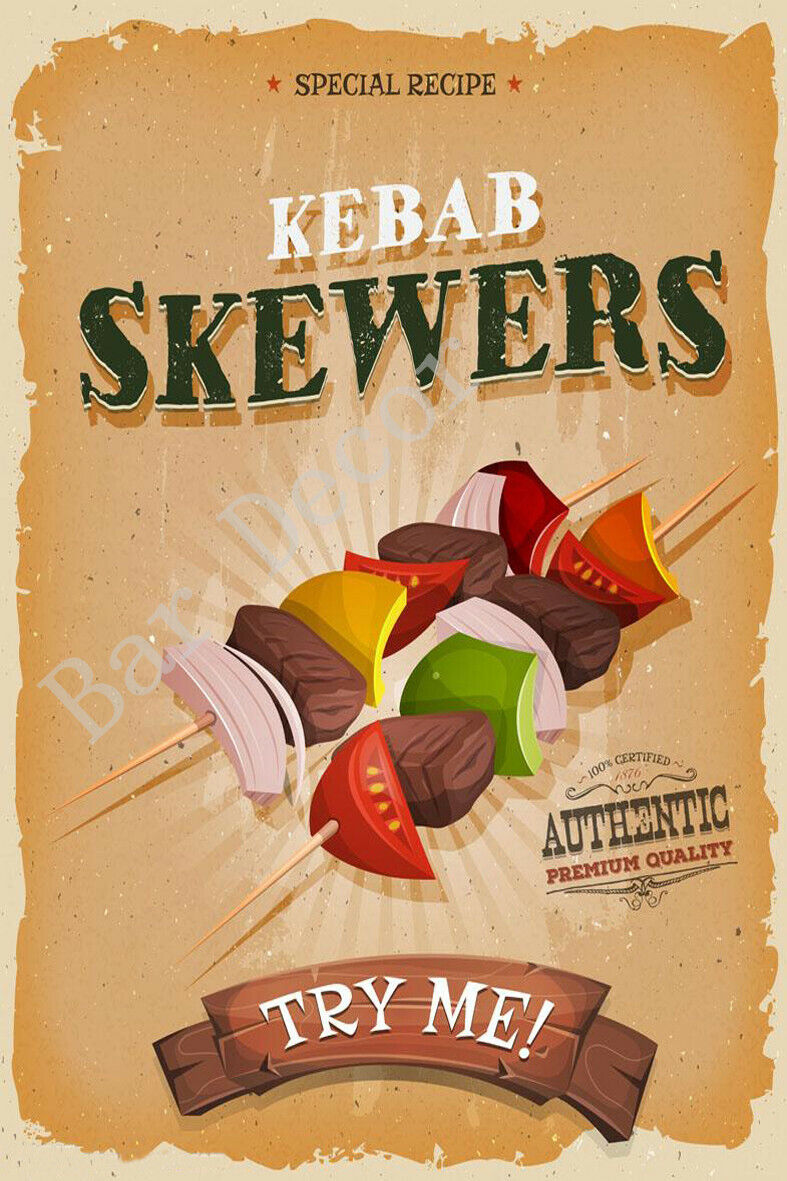The image is an advertisement styled like a vintage postcard with a worn, light brown background and an aged feel. It features a light yellow border framing a darker yellow interior. The top middle of the poster showcases the phrase "Special Recipe" in black letters flanked by red stars. Beneath that, "Kebab Skewers" is prominently displayed, with "Kebab" in white letters and "Skewers" in dark green. The central focus of the advertisement is two pictures of shish kebabs skewered with beef, onions, red and yellow peppers, green peppers, and tomatoes. On the right side, the text "100% Certified, Authentic, Premium Quality" emphasizes the craftsmanship of the recipe. Additionally, a subtle overlay of the phrase "Bar Decor" adds to the nostalgic charm of the image. At the bottom center, a small wooden sign with white letters invites viewers to "Try Me." This retro poster conveys a vividly detailed and enticing invitation to enjoy the authentic kebab recipe.